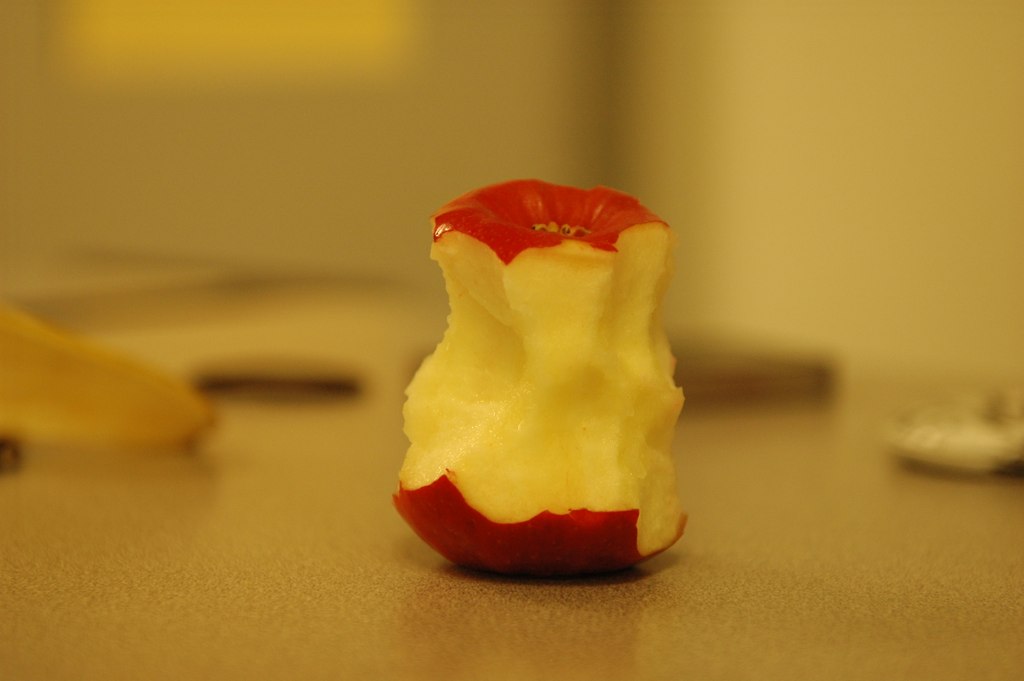A partially eaten apple, prominently positioned in the center of the image, dominates the composition. The apple's vibrant red skin is visible on the top and bottom, while the yellowish flesh is exposed in the middle where it has been half-eaten. Bite marks create irregular indentations and curves, giving the fruit an uneven, textured appearance. Surrounding the apple, the background is softly blurred, and indistinct objects on the table behind it fade into obscurity, ensuring that the viewer's attention remains fixed on the apple itself. The photograph captures the simplicity and detail of the everyday subject, emphasizing the contrast between the apple's bright exterior and its chewed, interior flesh.